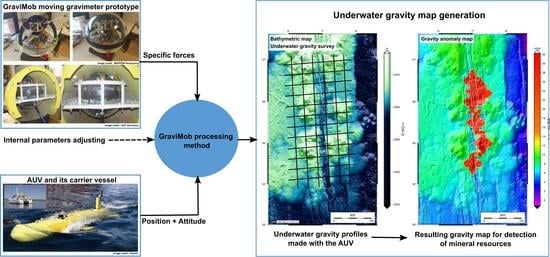The image is a comprehensive diagram titled "GraviMob Processing Method". On the left side, it features a series of four photos labeled "GraviMob Moving Gravimeter Prototype." These images depict a cylindrical object, with a transparent glass covering and a yellow frame around it. Accompanying this, the labels "Specific Forces" and "Internal Parameters Adjusting" are noted. Below this section is another diagram showing an "AUV and its carrier vessel," represented by a yellow submarine-like vehicle. There is an annotation for "Position plus Attitude," indicating its movement and orientation data feeding into the blue circle labeled "GraviMob Processing Method". This blue circle has arrows connecting to two additional images on the right side. These images illustrate "Underwater Gravity Map Generation," displaying two distinct mapping visuals. The left map shows a blue grid with checkerboard-like black lines, while the right map is a multicolored heat map, labeled "Gravity Anomaly Map," used to detect underwater mineral resources.